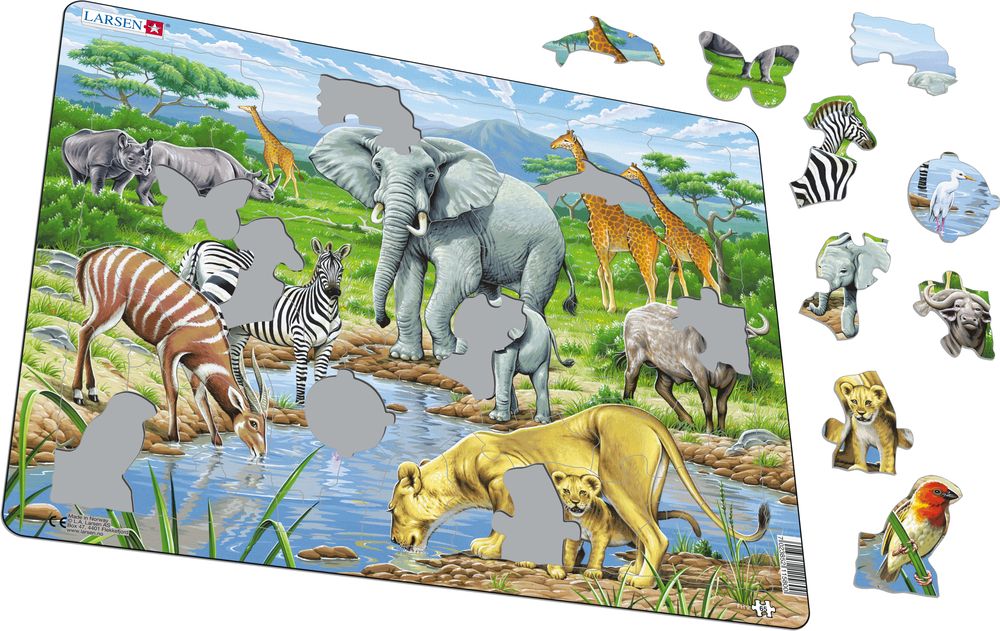This image features a colorful, illustrated children's puzzle set against a white background in landscape orientation. The subject is an African safari scene teeming with various wildlife, centered around a tranquil blue pond. The puzzle board, located on the left side of the image and angled with its short ends facing the top left and bottom right, is mostly assembled but has a few missing pieces that are arranged alongside its gray cardboard backing on the right side of the image.

The vibrant safari scene captures several animals: gray elephants with white tusks, black-and-white-striped zebras, a brown antelope with white stripes and two horns drinking from the pond, and a brown lion with a yellow mane and white underbelly alongside her cub. Additionally, there’s a graceful, spotted giraffe, a gray rhinoceros with a prominent horn, and a bird, possibly a crane or water buffalo bird. The surrounding environment is dotted with green-leaved trees typical of a safari landscape, green grass, darkish green mountains in the background, and a sky filled with blue hues and white clouds.

In the top left corner, there is a logo with the blue text "Larsen," next to a red square containing a white star. A black and white barcode is positioned in the bottom right corner of the image. The overall style of the illustration is realistic yet detailed, giving an impression of photographic representationalism as the puzzle appears to float seamlessly on the white backdrop.